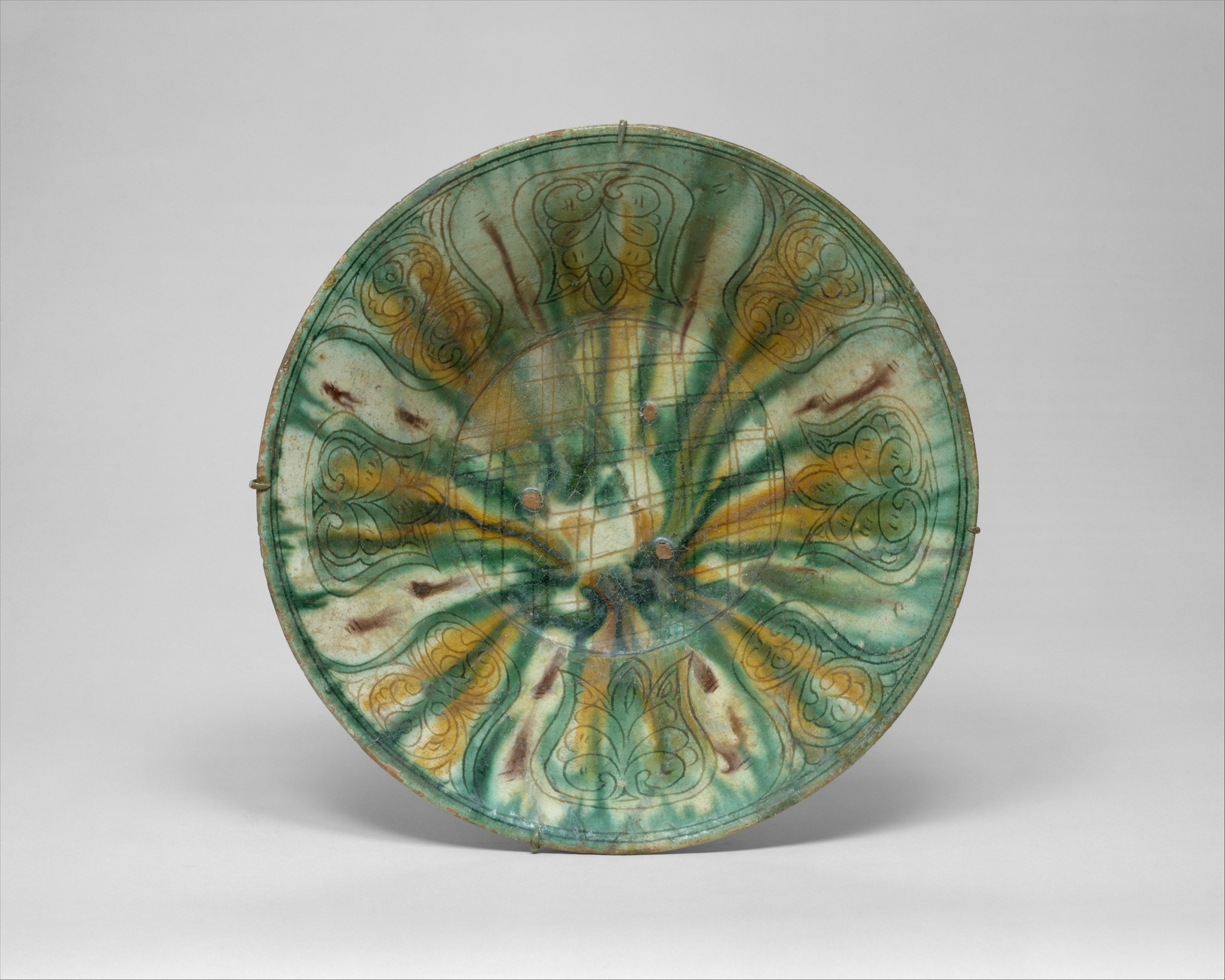The image showcases an old, ornate glass plate standing upright against a light gray background, likely supported by a stand with small silver brackets visible at the top, bottom, and sides. The plate itself features a green and brown motif with smeared strokes of paint intertwining mustard-colored streaks, creating an unstructured yet intriguing design. Along the edges, the paint appears chipped, adding to its vintage charm. The centerpiece of the plate is adorned with what resemble flower petals arranged in a circular pattern, contributing to its detailed, old-fashioned aesthetics. Amidst the abstract coloration, which includes shades of yellow, tan, and brown radiating outwards, the plate also exhibits a heavy green border and three distinct dots of color at its center. Additionally, a piece of dark gray cloth, which appears folded, lies beneath a dark gray, wiggly sperm-like figure with a solid charcoal-colored head, adding an unusual and unexpected element to the composition.